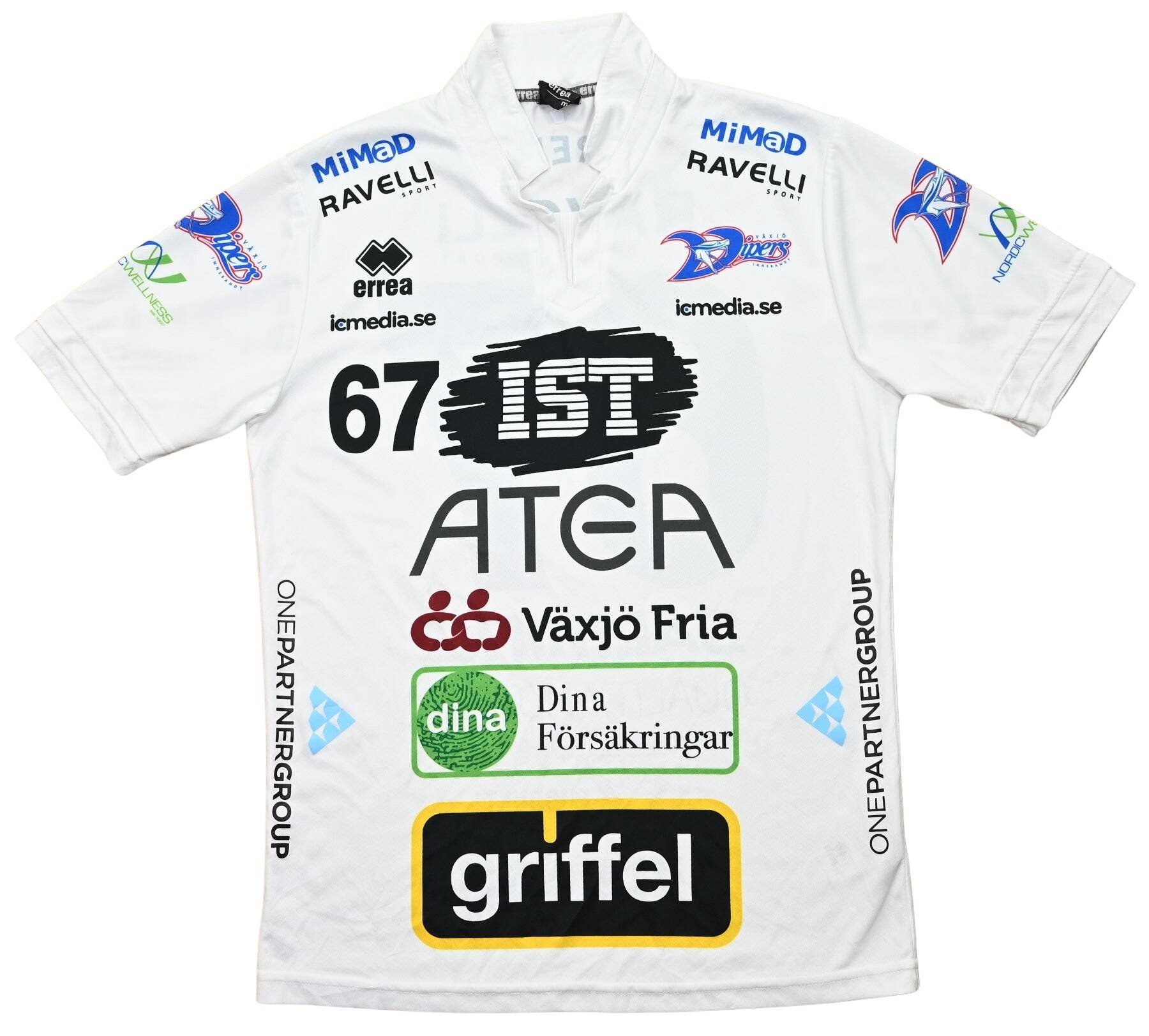The image features a white, short-sleeved, collared polo shirt, designed in a style reminiscent of European sports apparel, potentially for a soccer team. The shirt is heavily adorned with various advertisements and text in non-English languages, likely Norse or another Scandinavian language. Notable sponsors and logos include "67IST" and "ATEA" prominently displayed at the top. Below that, across the stomach area, are the words "Vaxjo Fria" and "Dina Försäkringar," with the latter inside a green circle on the right side. The left and right sides of the shirt under the arms feature vertically oriented "One Partner Group" text. Additional logos appear on both sleeves, notably "IEmedia.se" and "Errea." Another prominent ad is "Griffel," in white text on a black rectangle with a yellow outline. The shirt includes a mix of colors such as black, white, green, and blue, making the array of text and designs stand out clearly.